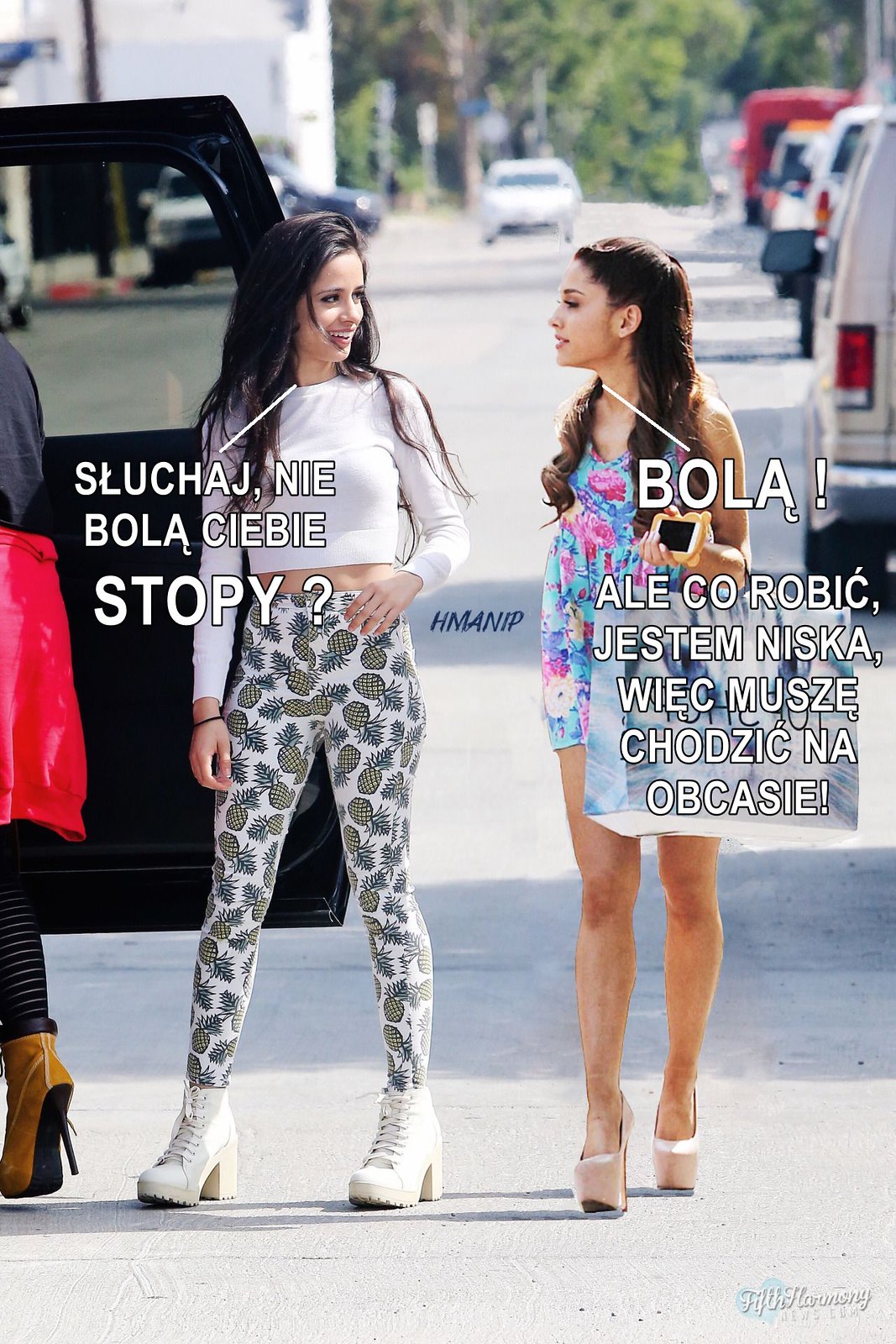In the image, we see three young women in a likely Eastern European setting, engaged in what appears to be an amused conversation. They are standing in the middle of the street next to an open door of a black van or truck. One woman is only partially visible; she is inside the vehicle, wearing a dark top, a red sweater tied around her waist, black striped tights, and camel-colored boots.

The other two women, standing outside the vehicle, are notably fashionable. The woman on the left has long, dark hair and is wearing a long-sleeved white crop top paired with white leggings adorned with a pineapple print and white platform boots. She seems to be engaging in conversation with the woman on the right, who also has long, dark hair. This woman is dressed in a very short blue and pink floral mini dress and is carrying a large shopping bag, suggesting a recent shopping trip.

There is dialogue written over the image in an unrecognizable language, adding a meme-like quality to the scene. The women's clothing and the open vehicle suggest a casual, perhaps spontaneous moment caught in the middle of an urban setting.